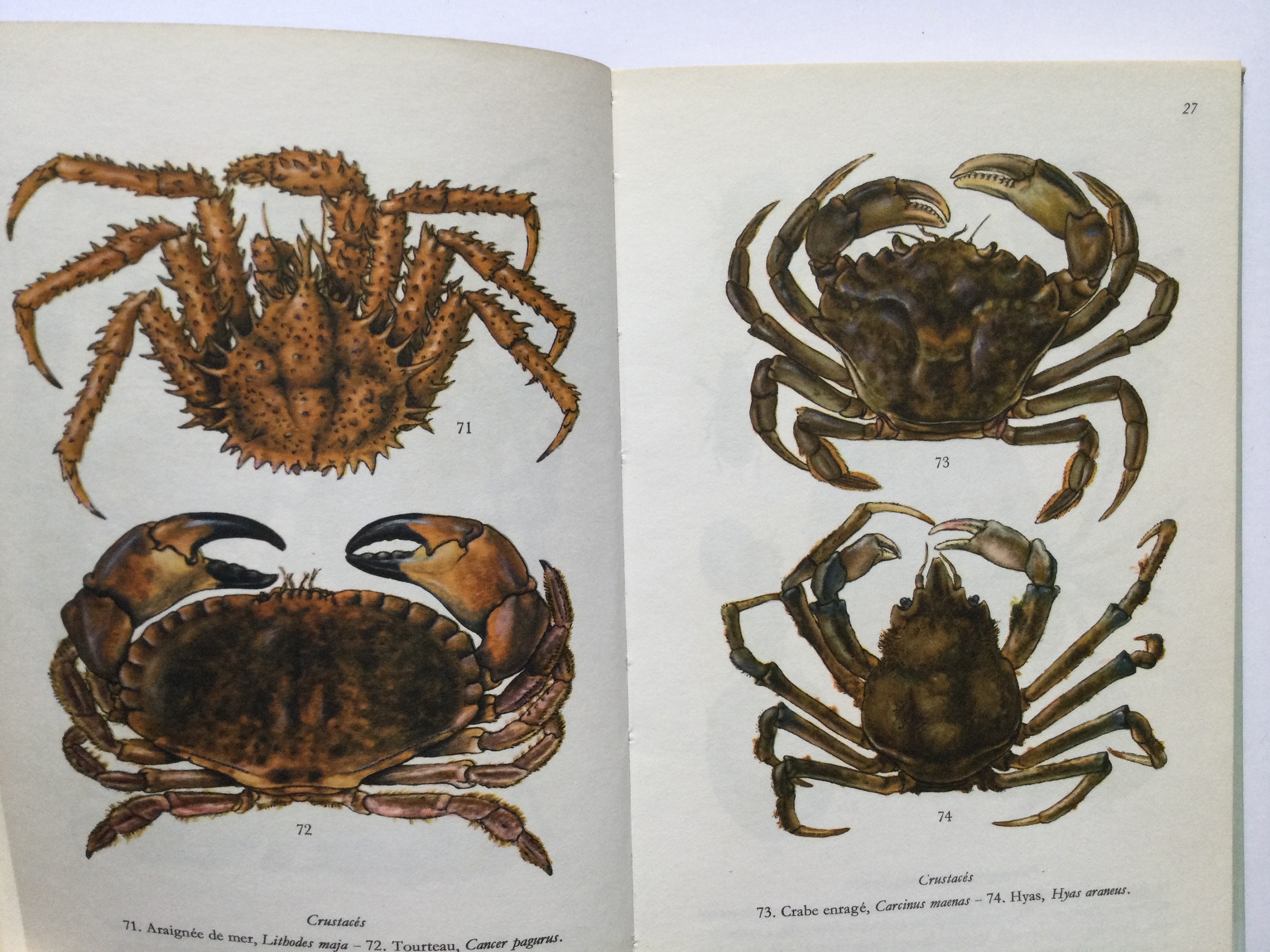The image captures an open book set against a very light blue, almost white background. The book features detailed and lifelike artistic illustrations of different types of crabs on facing pages, numbered 71 to 74. On the left-hand page, at the top, there is a brown crab with dark brown speckles (71), followed by a more conventional-looking brown pincher crab with black pinchers (72) beneath it. The right-hand page also displays two brown crabs; the upper illustration is labeled 73 and beneath it another crab is labeled 74. The specific names of the crabs are written underneath the illustrations in French, but only "Crab and Rage" for 73 and "Highest" for 74 can be discerned. The page number 27 appears in the upper right-hand corner of the right-hand page. The overall image is square, with the book's white pages contrasting against the light blue background, and it appears to have been photographed indoors using natural lighting.